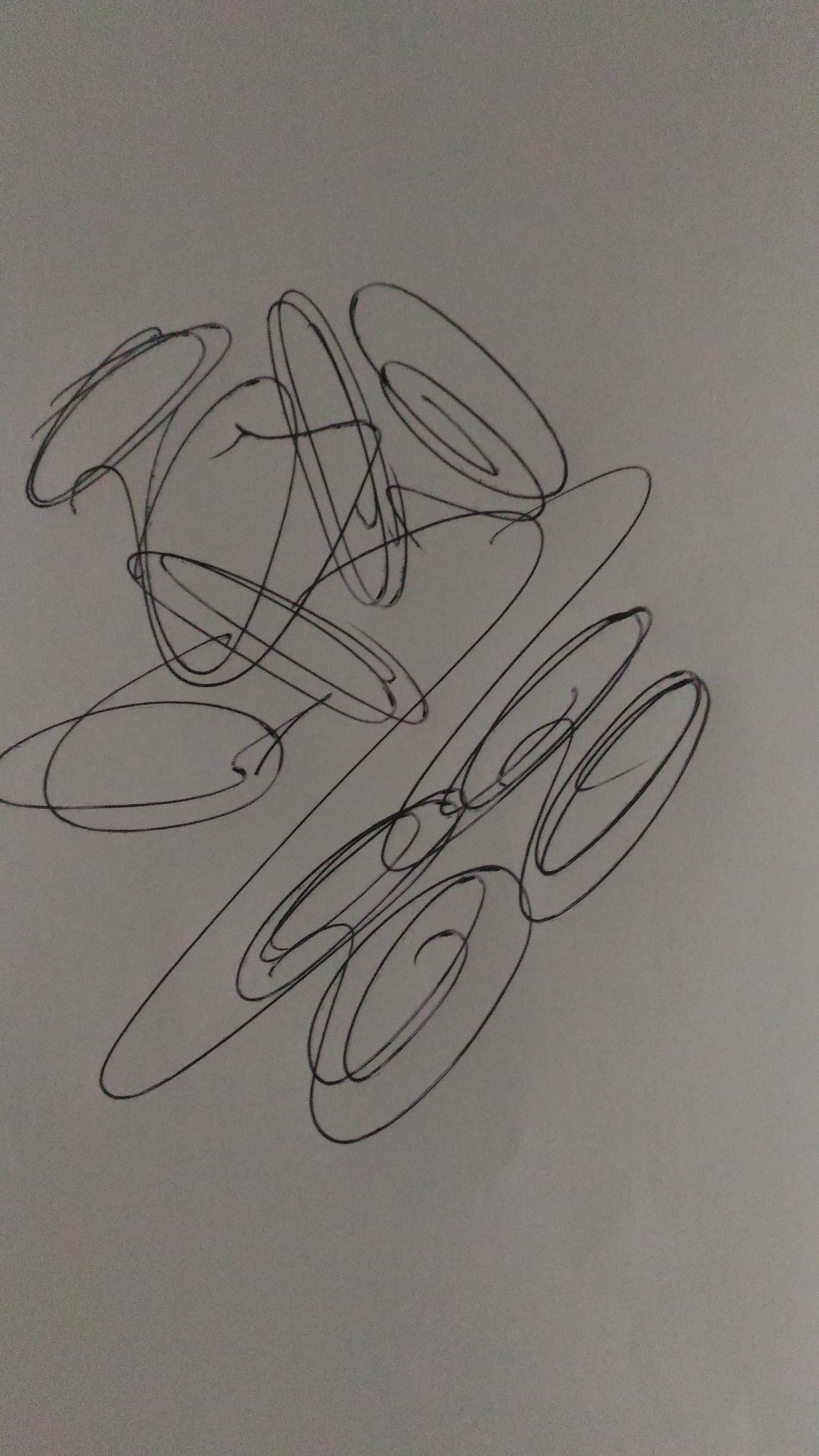The image features an intricate pattern of black squiggly lines on a white sheet of paper. The lines exhibit numerous curved and circular configurations, creating a dynamic and visually captivating composition. Towards the bottom of the image, a series of spiral shapes are arranged side by side, forming an hourglass-like pattern. Above each of these spirals, additional spiral shapes are drawn, echoing the design below. Two squiggly lines extend outward from this central grouping, first moving left, then curving right, and finally arcing upward slightly before veering left. These lines eventually intersect with another prominent spiral shape. To the left of this central spiral, two small circle shapes are present. Above the central spiral, there are two additional circle shapes with loose, short lines extending slightly to the left from them. At the bottom of the image, there is a U-shaped line, which features a branch extending from its right side, adding to the complexity of the overall design.